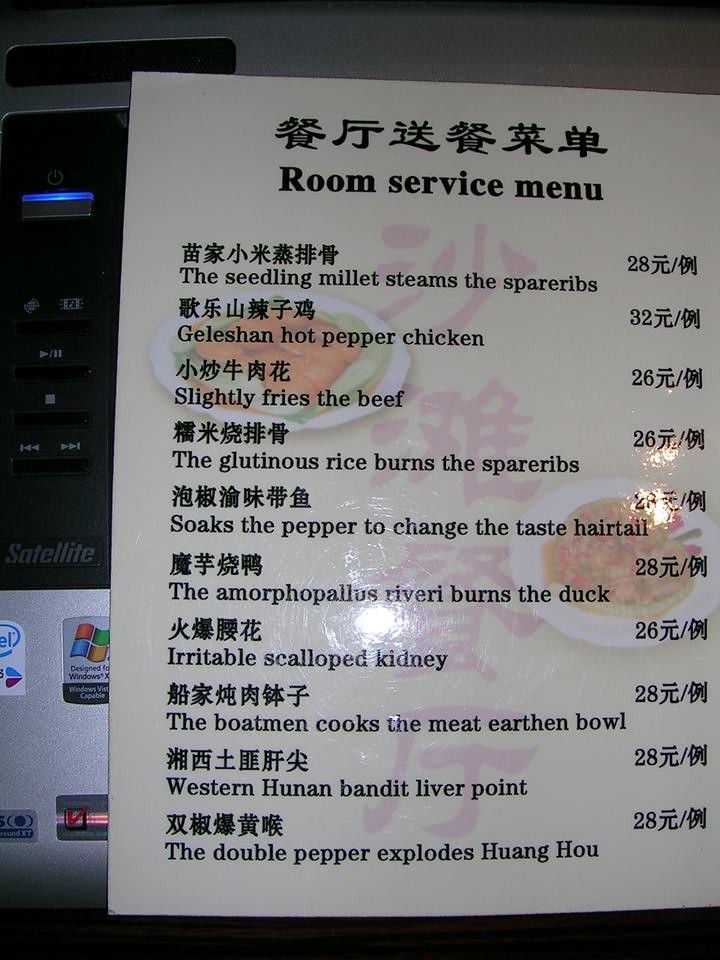This photograph showcases a bilingual menu, featuring both English and possibly Japanese text, held up in front of what appears to be a computer screen, as indicated by the visible logos in the background. The prominent title of the document reads "Room Service Menu." Here's a detailed list of the items on the menu along with their respective prices:

1. Seedling Millet Steams the Spare Ribs - 28
2. Gishan Hot Pepper Chicken - 32
3. Slightly Fries the Beef - 26
4. The Glutinous Rice Burns the Spare Ribs - 26
5. Soaks the Pepper to Change the Taste - Hair, Tail (Price unreadable)
6. The Amorphous Rivery Burns the Duck - 28
7. Irritable Scalloped Kidney - 26
8. The Boatman Cooks the Meat Earthen Bowl - 28
9. Western Hoonin Bandit Liver Point - 28
10. The Double Pepper Explodes (Unintelligible) - 28

The peculiar and amusing translations suggest that this menu could either be the result of a translation error or a playful jest.